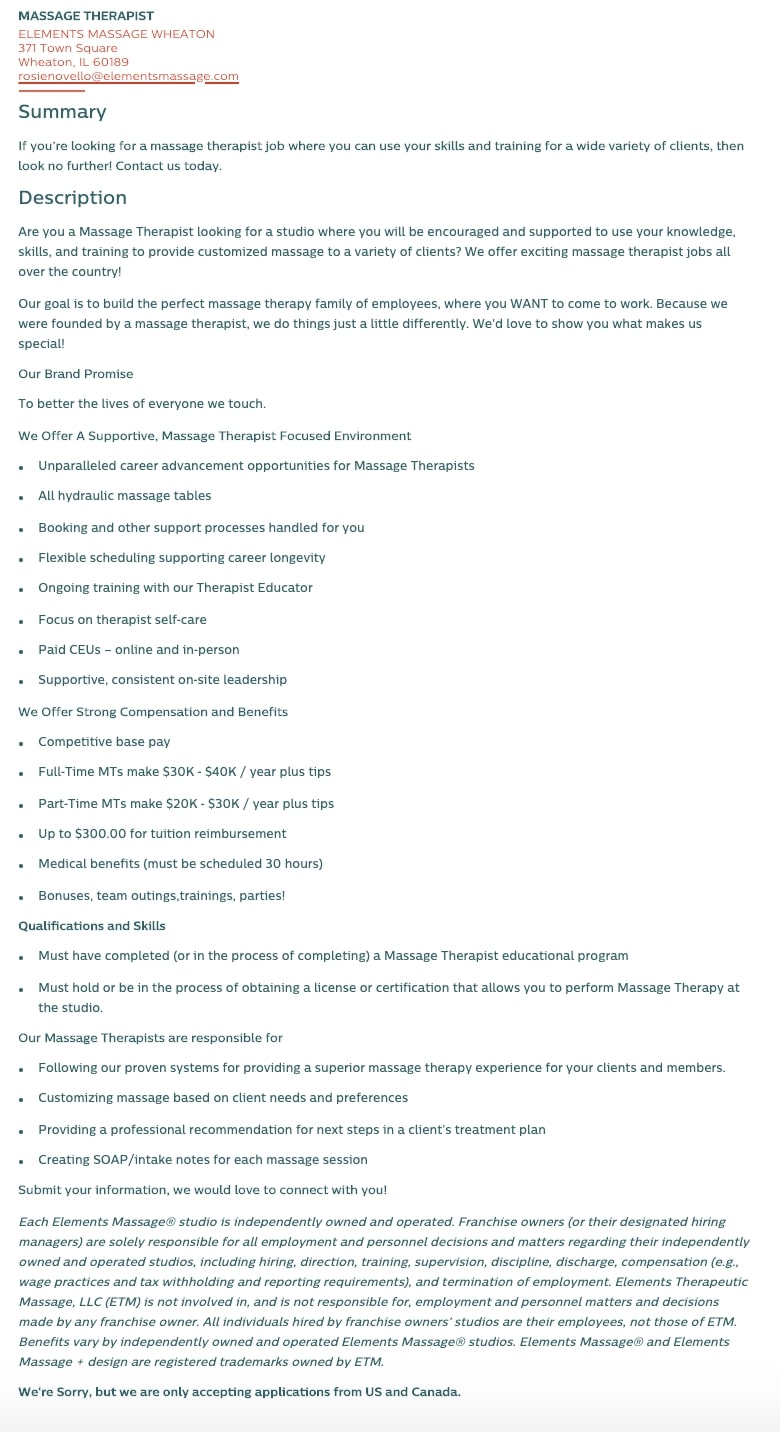The image is a screenshot of a long webpage with very small text, making it difficult to read. The header in the upper left corner reads, "Massage Therapist, Elements Massage Wheaton, 371 Town Square, Wheaton, Illinois, 60169." Directly below that, there is an underlined email or website address, but the text is too small to decipher.

The main body of the website features very small green text. At the top, there is a section that begins with a summary stating: "If you're looking for a massage therapist job where you can use your skills and training for a wide variety of clients, then look no further. Contact us today."

Underneath this summary is a description that reads: "Are you a massage therapist looking for a studio where you would be encouraged and supported to use your knowledge, skills, and training to provide customized massage to a variety of clients? We offer exciting massage therapist jobs all over the country."

Beneath this, there is a header stating, "We offer a supportive massage therapist focused environment." Following this header, there are over a dozen bullet points listing the various benefits and opportunities provided by the studio.

This detailed caption provides a comprehensive overview of the image content while addressing the main sections and key information despite the difficulty in reading the text due to its small size.